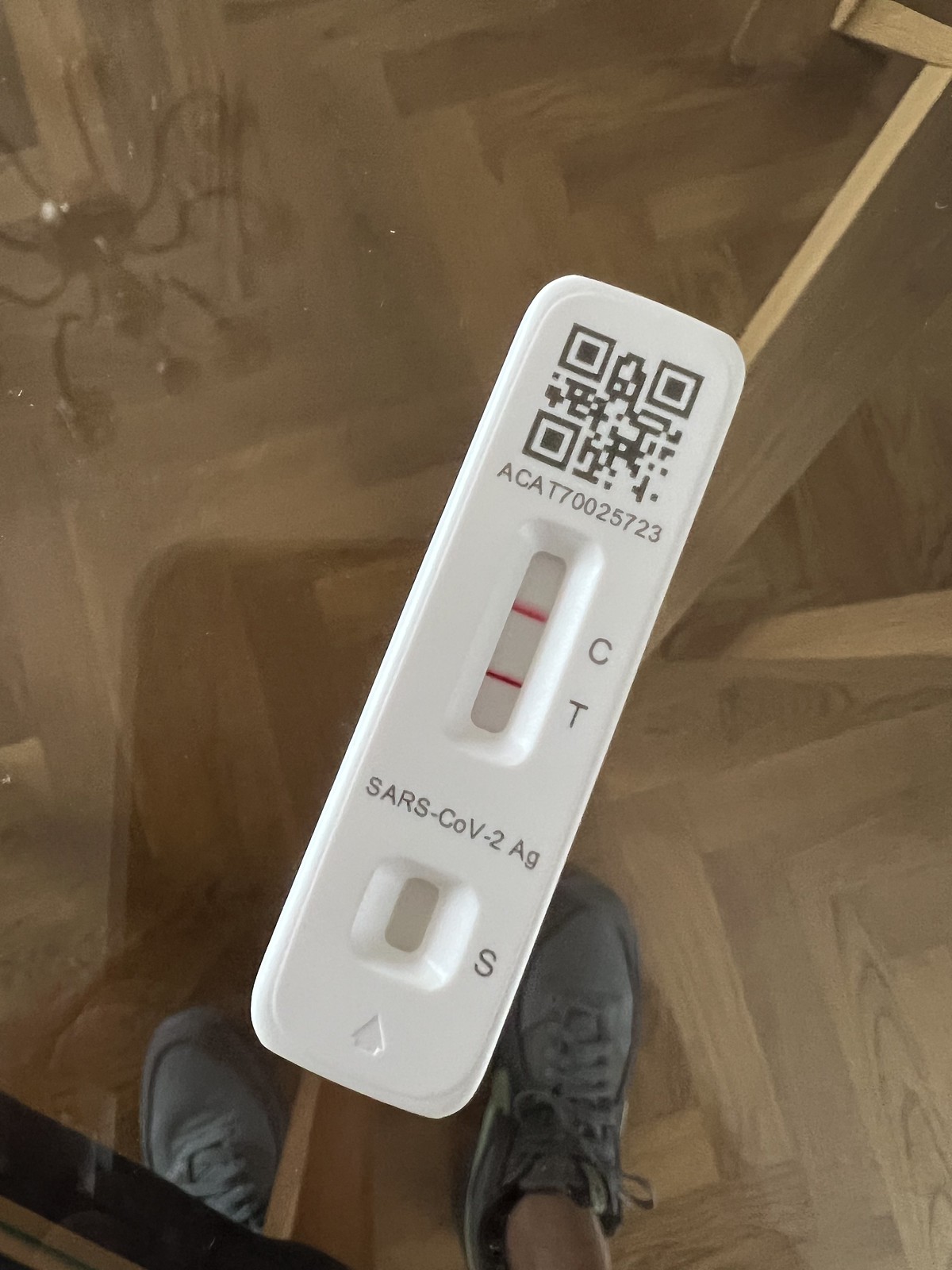The image features a COVID-19 test strip prominently displayed on a glass table. The test strip is white and at the top, it displays a barcode labeled "ACAT 70025723" in black text. Below the barcode, there are red lines corresponding to the "C" and "T" markers, which indicate the test results. The strip is labeled "SARS COV2AG" right above the "S" at the bottom of the test.

In the lower portion of the image, you can see a pair of black Nike tennis shoes, identifiable by the iconic stripe on the left shoe. The floor beneath the table consists of brown bits, adding texture to the scene. To the left, a chandelier is partially visible, contributing to the ambiance. Also captured within the mirrored surface of the glass table is the reflection of the photographer's phone.

On the right side of the image, some wooden supports that likely belong to the table frame can be seen, reinforcing the setting of the shot being taken through a glass surface.